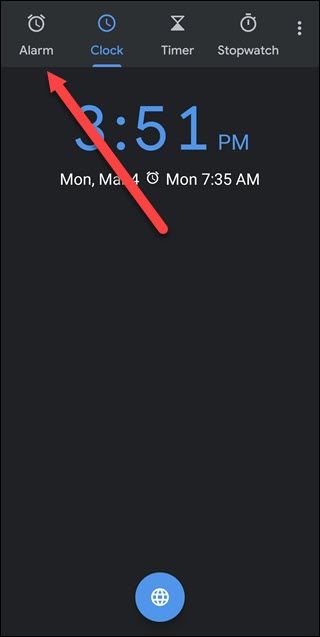This image is a screenshot of a clock app on a mobile device. The background is predominantly black, enhancing the overall contrast and clarity. 

At the top, there is a dark gray bar featuring several selectable tabs. From left to right, these tabs include: an alarm clock icon paired with the word "Alarm," a clock icon next to the word "Clock" (which is highlighted in blue with an underline indicating it is the active selection), an hourglass icon labeled "Timer," a stopwatch icon labeled "Stopwatch," and a three-dot menu icon for additional options.

Below this bar, in blue text, the current time is displayed as "3.51 p.m." and the date as "Monday, March 4th." An alarm icon is shown beneath, with a set alarm time of "Monday, 7.35 a.m."

At the bottom of the screen, there is a prominent blue circular button featuring a white globe symbol.

Superimposed on this layout is a long red arrow pointing towards the 'Alarm' tab at the top, suggesting attention or interaction with that specific function.